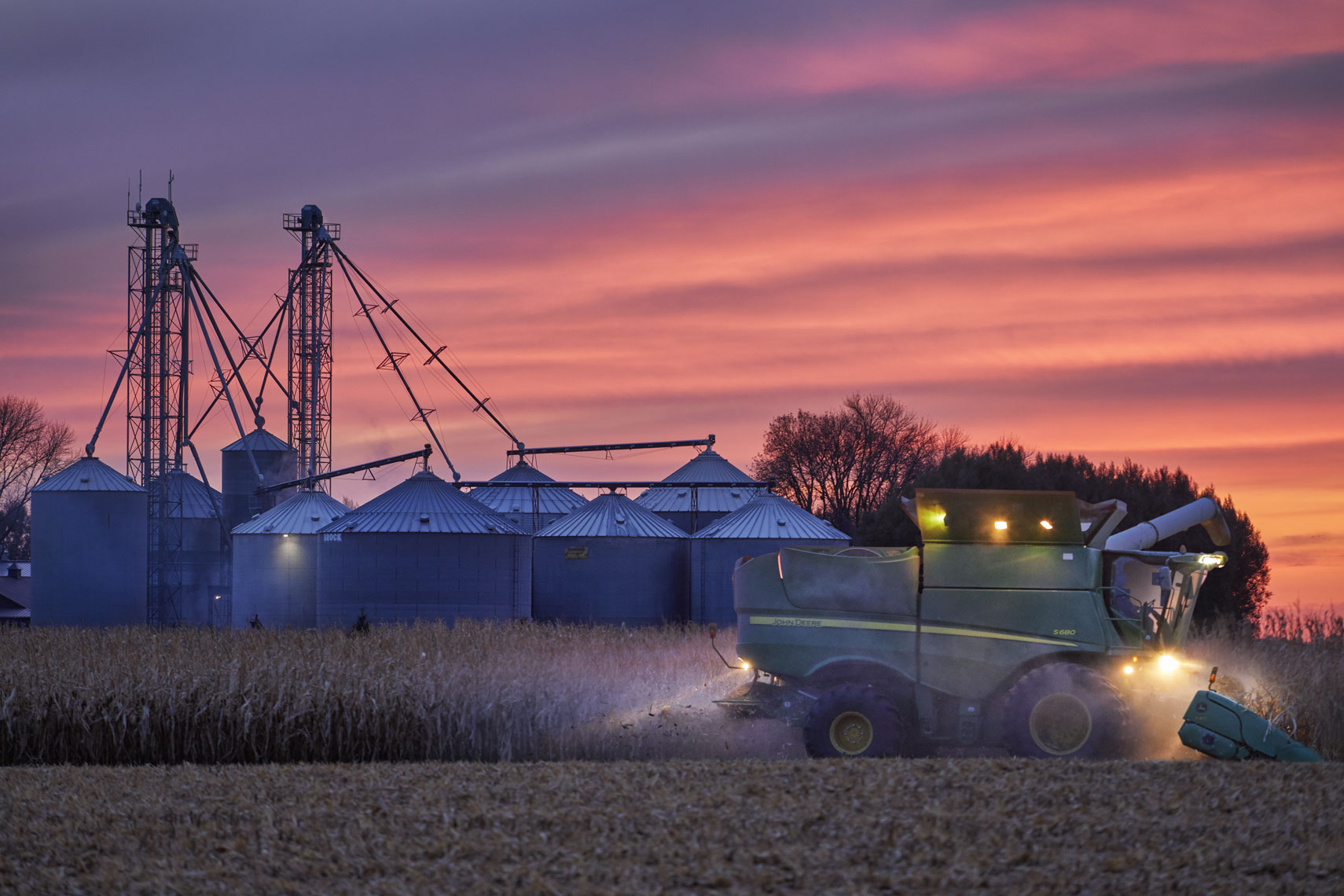The image, captured at dusk, showcases a serene farming scene under a stunning sky transitioning from pink to dark purplish-blue. Dominating the right foreground of the picture is a green combine harvester, with its lights on, collecting grains in what appears to be a wheat field. The harvester, equipped with large black wheels, moves against a backdrop of tall, silhouetted trees, which appear black due to the dim light. In the background, silver grain silos rise into the twilight, with tower-like structures that extend upwards, and additional towers can be observed to the left. The overall ambience is set by the almost-set sun, casting a soft purple haze over the scene, creating a tranquil and picturesque atmosphere.